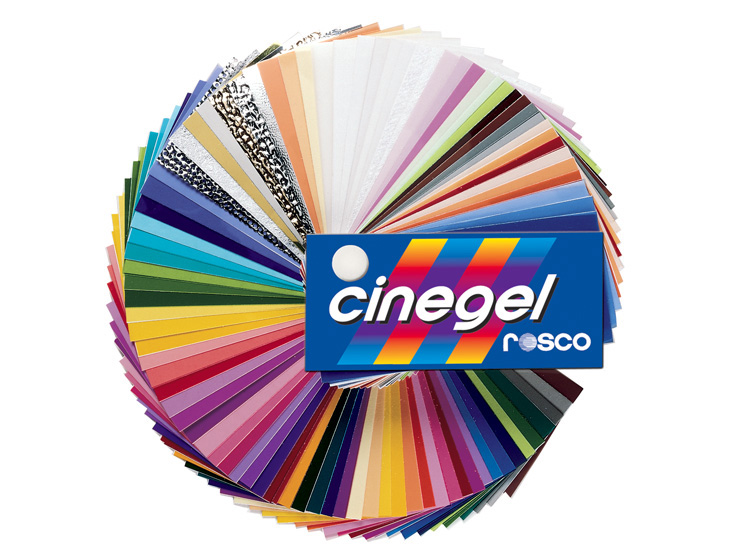The image showcases a comprehensive sample palette from Rosco's Cinegel collection, featuring a broad spectrum of colors for various applications. The central hub, where the shades converge, prominently displays the brand name "Cinegel" and "Rosco," each in bold, uppercase letters next to the company's logo. The palette includes an array of hues such as multiple shades of white, mauve, greens, yellows, purples, blues, and oranges. While there are fewer variations of pinks and reds, the collection offers some textured options in black and white patterns. Blues are well-represented, accompanied by several tones of green and an extensive range of purples, making it a versatile tool for color selection.